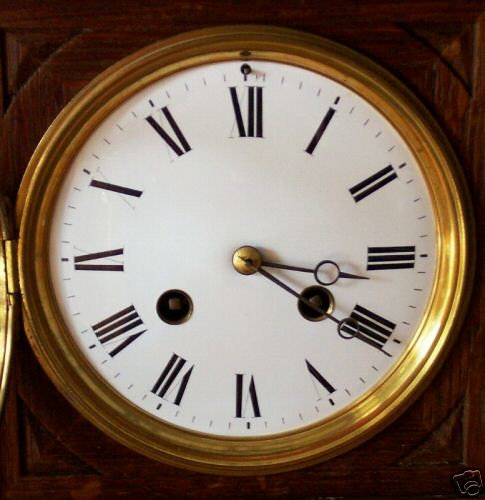This image showcases a close-up of a classical, large clock face, suggesting it might be part of a grandfather clock. The clock has a white face encased in a brass or gold metallic frame. Its time shows 3:21. The clock features prominently black Roman numerals for its numbers. The distinctive metal hands, both the hour and minute hands, are slender with pointed ends and feature circular details near their centers, secured by a gold button. On the clock face, there are two small black dots, each containing two squares, located above the four and eight o'clock positions. The clock is set against what appears to be a wooden frame, likely oak or dark reddish-brown, adding to the vintage aesthetic. The door or cover of the clock, which is hinged on the left and partially open, is also made from brass. On the lower right of the image, a white object is partially visible, set against the dark wooden structure. The overall craftsmanship and design elements suggest this clock is a grandfather clock with detailed woodwork including small triangular cutouts at the corners.